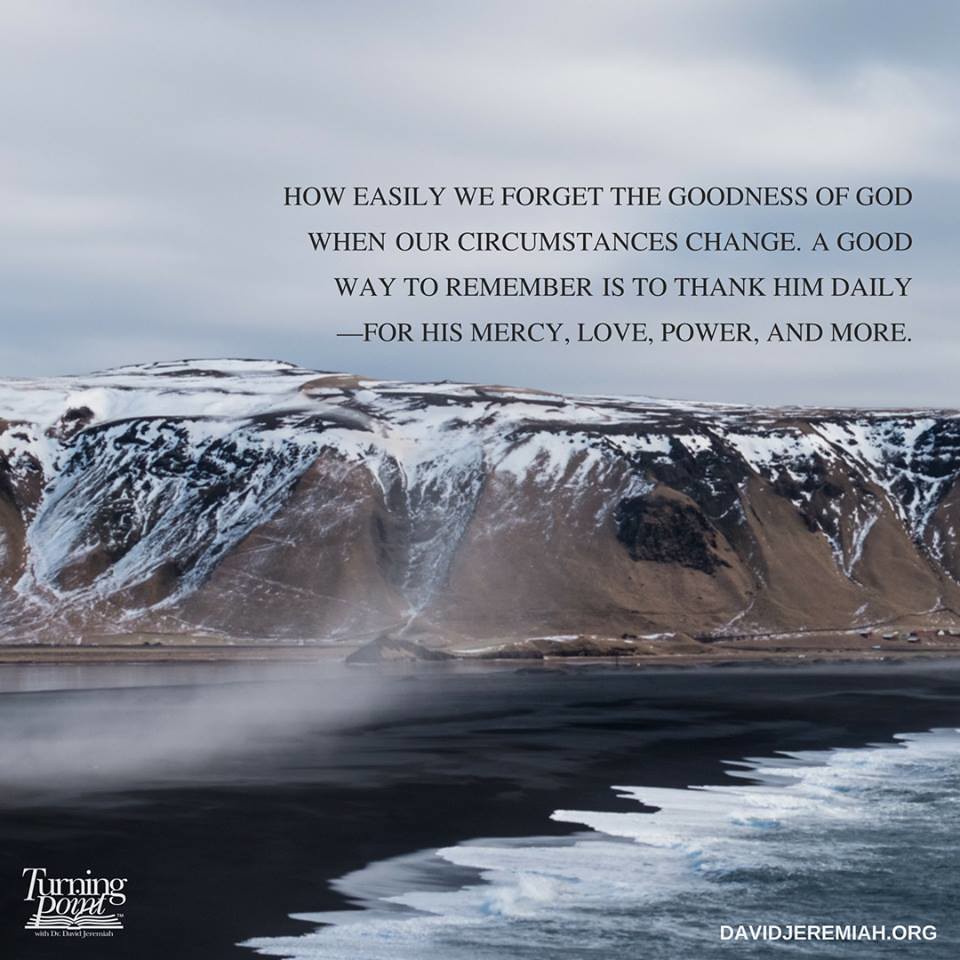The image is a square photograph depicting a dramatic Arctic landscape with a high contrast between the icy forewaters and the towering, snow-capped mountain peaks in the background. In the lower right corner, a watermark reads "davidjeremiah.org," and in the lower left corner, "Turning Point" appears in white text, accompanied by a book icon. The bottom right also shows a shoreline where white foamy waves crash against what appears to be either dark sand or deep, dark blue water. The steep mountain cliffs, dark brown and adorned with patches of foliage, rise sharply to meet the flat, snow-covered ridgeline. The sky above is predominantly gray with dark clouds, and across it runs a poignant message in black text: “How easily we forget the goodness of God when our circumstances change. A good way to remember is to thank Him daily for His mercy, love, power, and more.”